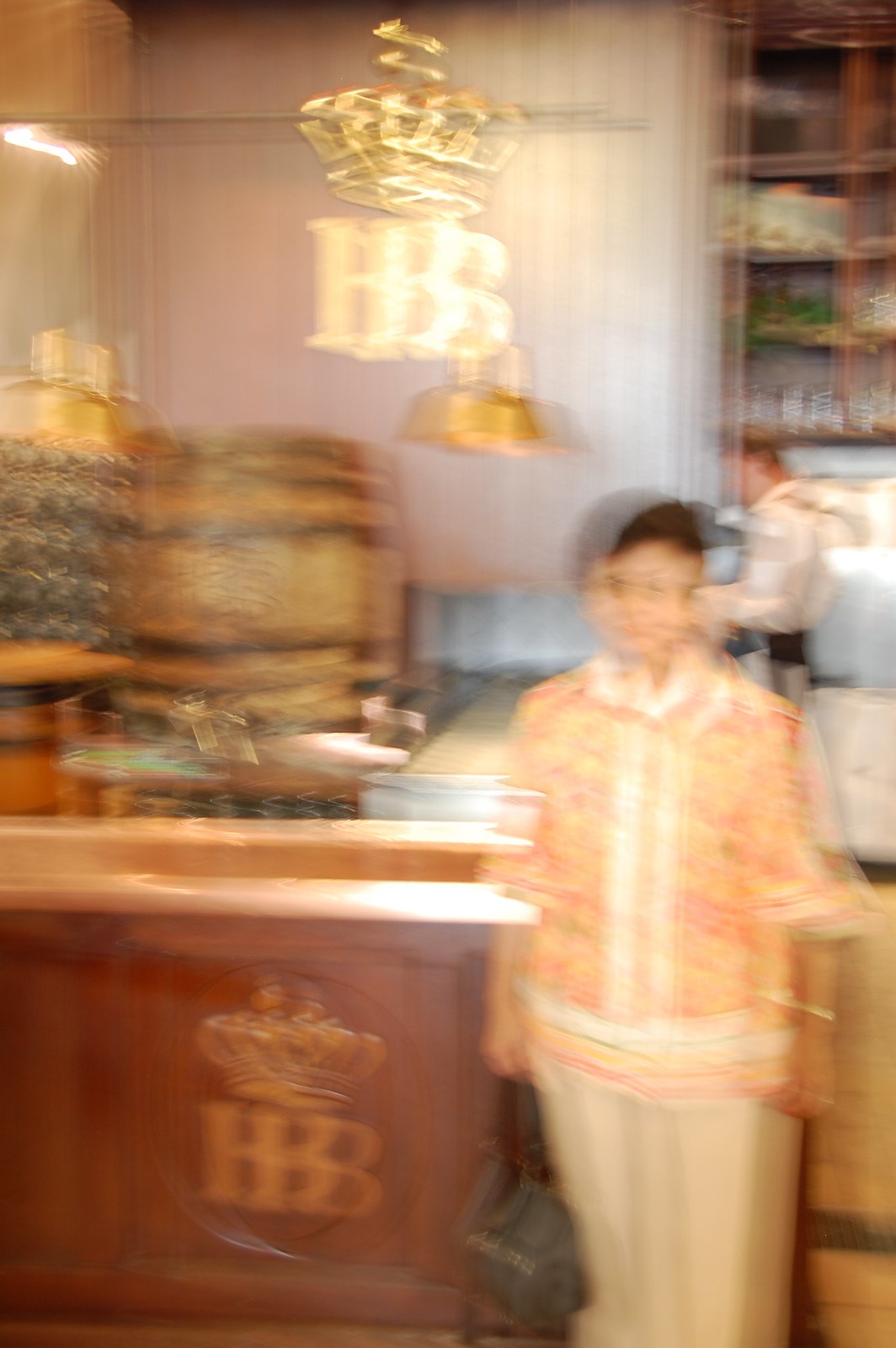In this blurry photograph, an Asian woman stands facing the camera. She is dressed in pleated, cream-colored slacks that are loose-fitting, paired with a tunic top adorned with a floral pattern in shades of orange and white. The tunic features a white border along the buttons in front and at the cuffs, which end just above her elbows, and it is completed with a white-collared neckline. The woman has short, dark hair and is wearing glasses. Draped over her shoulder is a gray purse with a brown strap. She is positioned next to a counter that prominently displays the letters 'HB' in gold, topped with a crown logo.